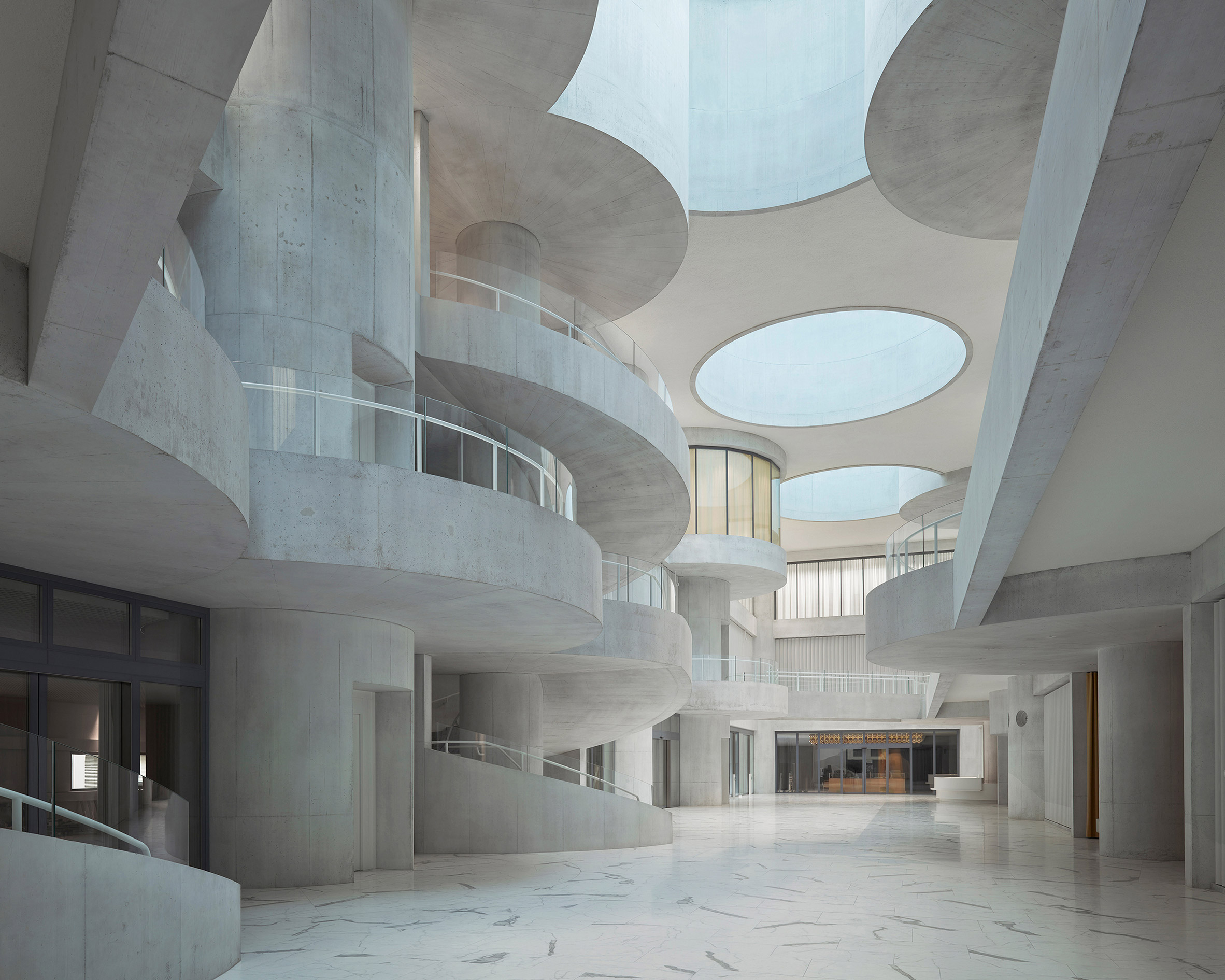The image captures the inside of a large, architecturally striking building that evokes elements of both a mall and an office space with its grand design. The structure features a long, marbled hallway with white floors accentuated by grey lines. Multiple floors are visible in the image, each with semi-circular glass balconies and rounded columns that ascend through the levels. The architecture has a brutalist influence, with white stone or concrete material showing grey division lines and some staining.

On both sides of the hallway, there are doors that could be entrances to stores or offices. The bottom left corner shows a stairway or railing, while staircases can be seen leading up to each floor. The building also boasts several circular sunroof panels in the ceiling, allowing natural light to pour in, creating an open, airy feel despite being indoors. The left-hand side features double doors and black-framed windows, whereas the right side, past one of the prominent columns, reveals a light brown door. Further down the hallway, there are more double doors, glass windows, and a large desk visible behind them. The overall aesthetic is enhanced by the rounded designs and a grand, open atmosphere, making the space as functional as it is visually appealing.